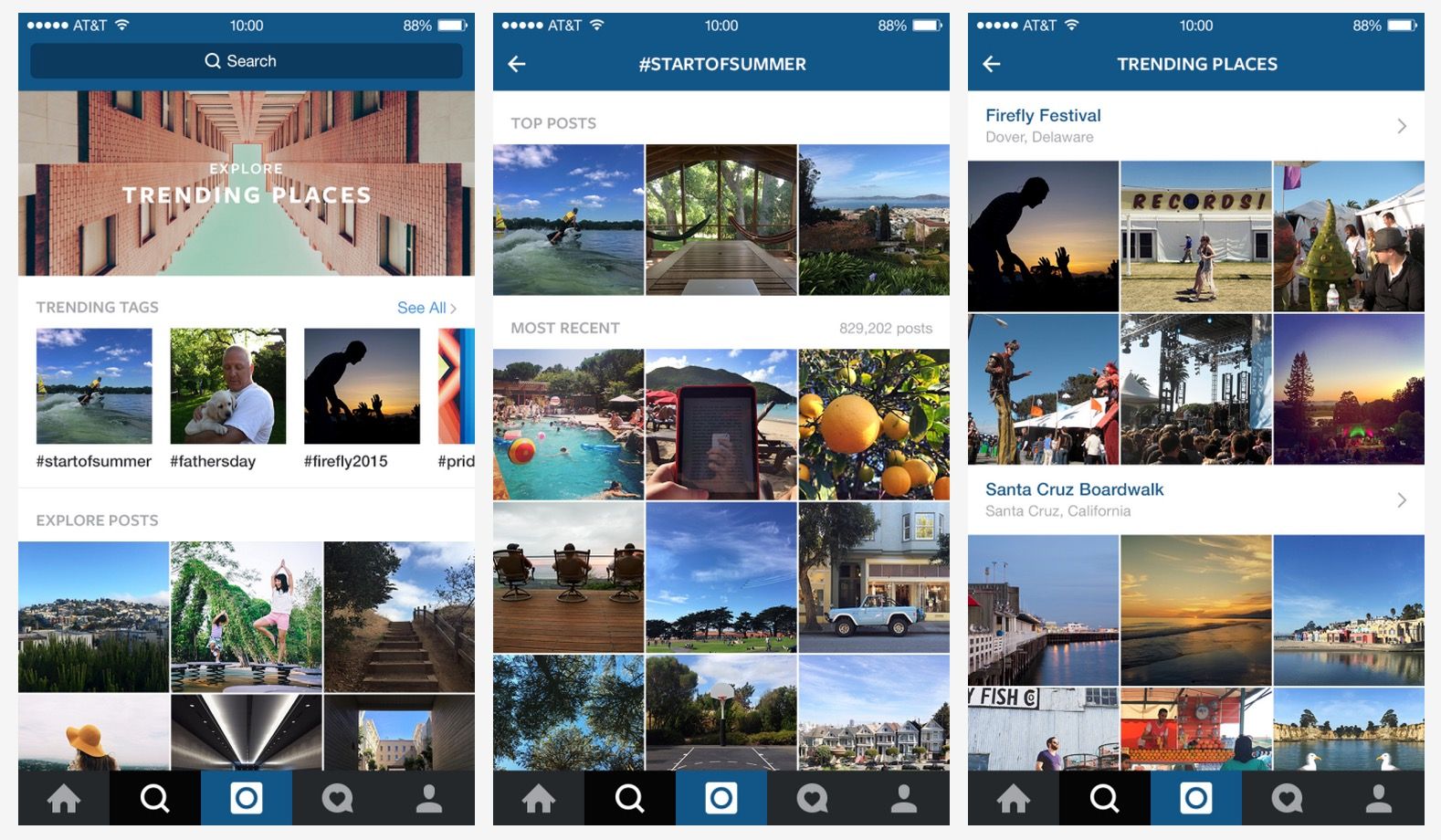The image is a screenshot compilation comprised of three smartphone displays, each illustrating sections of what appears to be a social media application. All three screens display a blue banner at the top, which includes the AT&T network identifier, Wi-Fi signal icon, a 10:00 AM timestamp, and an 80% battery indicator.

### Panel 1:
The first panel features a search bar prominently at the top, represented by a white magnifying glass icon and the word "Search" with a capital 'S'. Below the search bar, a section labelled "Explore Trading Places" is displayed, followed by trending tags such as "#StartOfSummer", "#FathersDay", "#Firefly2015", and "#Pride". Underneath, a segment titled "Explore Posts" showcases six different preview images from various posts. At the bottom, the navigation bar includes five icons: a house (home), a magnifying glass (search), a camera (new post), a heart (likes), and a person (profile).

### Panel 2:
The second panel is structured similarly at the top but introduces a hashtag section: "#STARTOFSUMMER" with a back arrow icon on its left. Below this header, two tabs display "Top Posts" and "Most Recent Posts", indicating there are 829,202 posts under this tag. The navigation bar mirrors the first panel with identical icons.

### Panel 3:
The third panel is headed by the phrase "Trending Places" and provides additional location-specific tags. It highlights "Firefly Festival, Dover, Delaware" alongside six representative images, followed by "Santa Cruz Boardwalk, Santa Cruz, California," again accompanied by six images. The bottom navigation bar remains consistent with the previous panels, showcasing the house, magnifying glass, camera, heart, and person icons.

Each panel visually organizes and presents distinct yet interconnected components of the app, indicating a seamless and intuitive user experience.